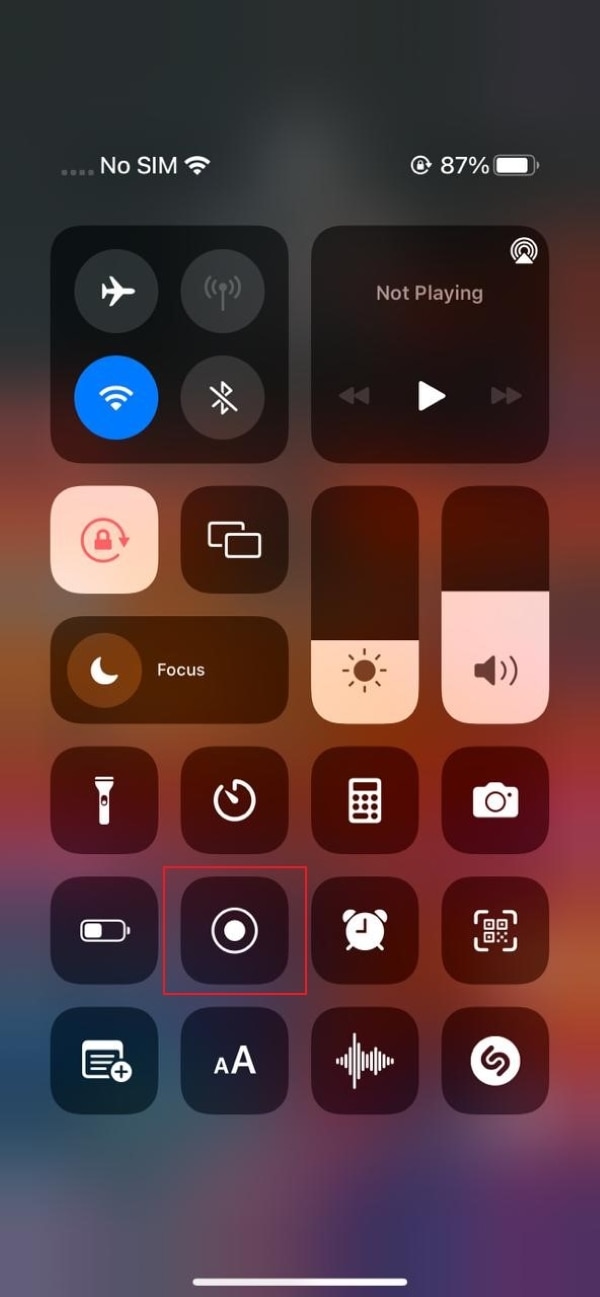The image depicts a smartphone screen showcasing an application with various functional icons. At the top of the screen, the status bar indicates "No SIM" alongside the Wi-Fi signal strength and a battery level of 87%. Also visible are the Bluetooth and Wi-Fi symbols, and indicators for Airplane Mode. Below the status bar, there's a range of clickable icons including controls for playing music, locking the phone, adjusting volume, and toggling the flashlight. Additionally, there are buttons for setting alarms, accessing the calculator, launching the camera, and powering off the device. This selection of icons is illuminated, organized into a user-friendly interface, and displayed clearly against the app's background.